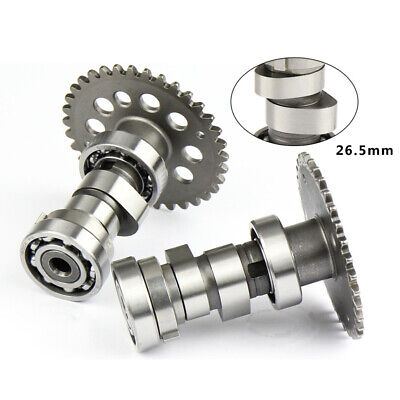The image depicts a detailed engineering diagram, likely from an instruction manual, featuring two silver gears set against a white background. The gears, designed to fit into a larger machine, are shown in two different orientations: one gear is positioned diagonally with its head facing the top right, and the other is almost horizontal but slightly tilted upwards, with its gear head facing right. Each gear features seven punched-out circular holes and is attached to a cylindrical metal shaft, embellished with multiple rings and bearing sections. The top right corner of the image includes a magnified inset, providing an up-close view of the gear details and highlighting the measurement "26.5 millimeters," indicating the size of the components. The gears, composed of stainless steel with varying light and dark tones, are precision-engineered to facilitate movement within a mechanical system.